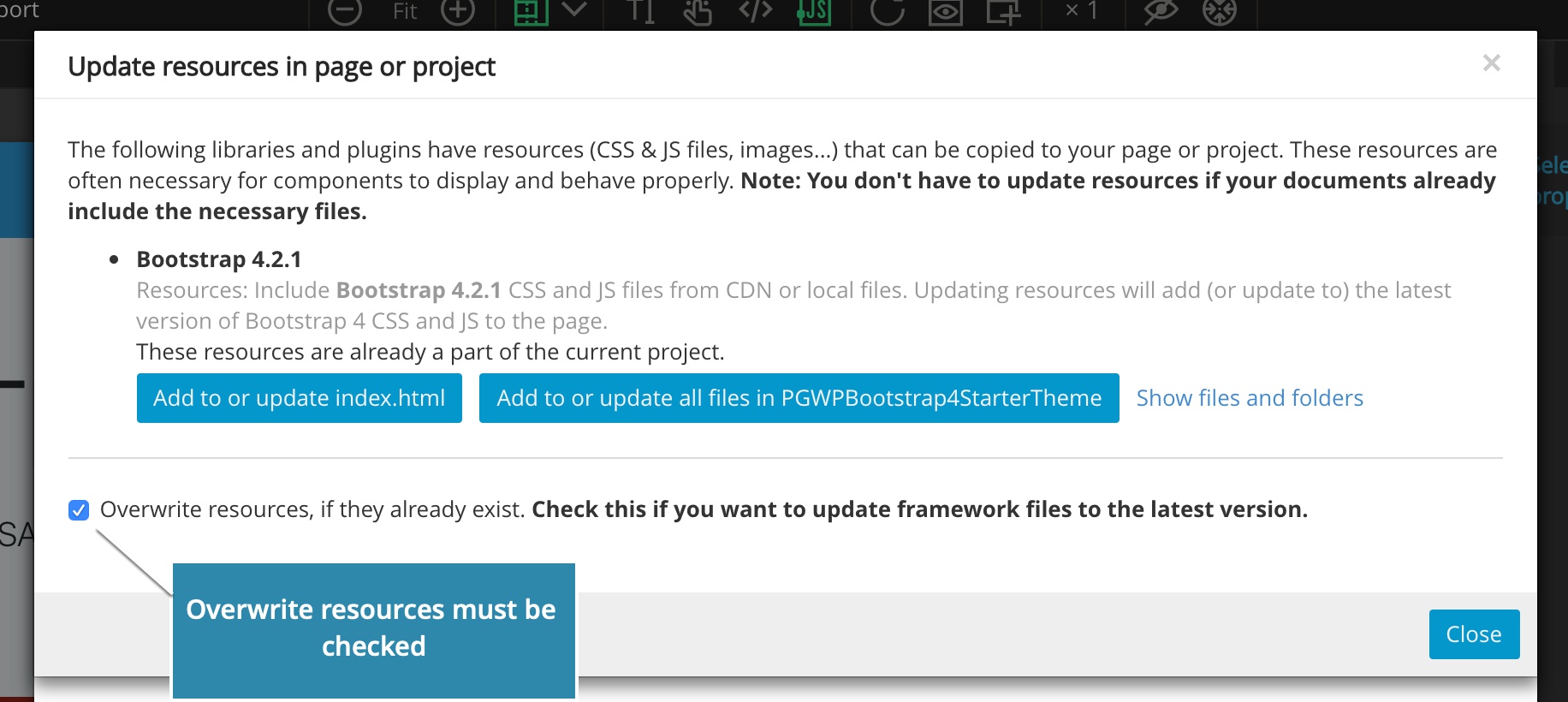This is a horizontal rectangular image predominantly featuring a white section overlaying a computer-generated background. In the top left corner of the white section, bold black text reads, "Update resources in page or project." Below this, in standard black text, it says, "The following libraries and plugins have resources (CSS and JS files, images) that can be copied to your page or project. These resources are often necessary for components to display and behave properly."

Next, a bold black note emphasizes, "Note: You don't have to update resources if your documents already include the necessary files."

Indented and marked with a bullet, "Bootstrap 4.2.1" appears in bold black text. Below this, in light gray lettering, it reads, "Resources: Include Bootstrap 4.2.1 CSS and JS files from CDN or local files. Updating resources will add (or update) the latest version of Bootstrap 4 CSS and JS to the page." An additional note in black text states, "These resources are already a part of the current project."

Toward the bottom, there are two horizontal rectangular buttons in turquoise with white text. The smaller button to the left states, "Add to or update index.html," while the larger button to the right reads, "Add to or update all files in PGWP Bootstrap 4 Starter Theme." Directly beside these buttons, turquoise text says, "Show files and folders."

At the very bottom, a small blue rectangular box with a white check mark features black text: "Overwrite resources if they already exist." Next to it, bold black text reads, "Check this if you want to update framework files to the latest version."

Beneath this, a darker turquoise horizontal rectangle with bold white lettering insists, "Overwrite resources must be checked." A diagonal line extends from the top left edge of this box to the smaller turquoise box containing the white check mark. Finally, at the bottom right, a small turquoise box with the word "Close" in white letters is displayed.